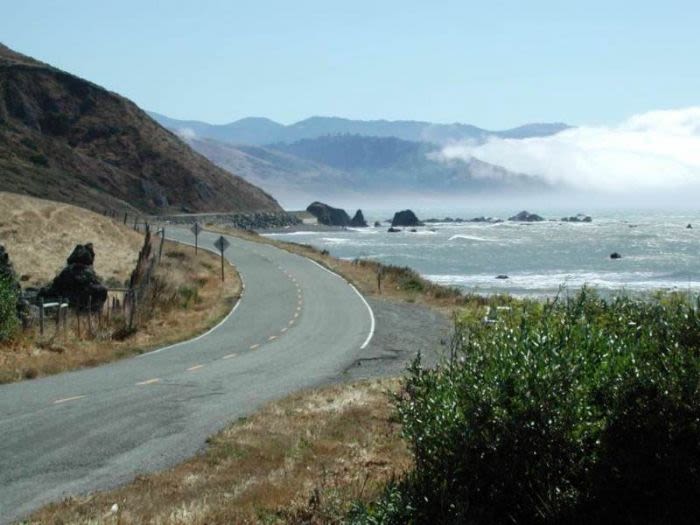This photograph, taken outdoors under the sun, captures a scenic coastal road winding its way through a picturesque landscape. The two-lane road starts from the bottom left corner of the image, curving towards the center and then back to the left, marked by a yellow dashed line and white edge markings. On the left side of the road, a wooden fence lines the edge along with several street signs shaped like rhombuses on tall poles. The shoulder of the road is light brown with grassy mountains and a few scattered shrubs.

To the lower right of the image, a shadowy green bush appears, flat-topped and casting a dark shadow at its base. Adjacent to this bush, the sea is visible, with blueish-gray waves crashing against the rocky shore. The horizon reveals more of the ocean stretching towards the middle right of the scene.

The backdrop of the photograph showcases a dramatic expanse of mountains—tall, brown peaks to the left and dusky blue mountains with low-lying clouds on the right, creating a striking contrast against the clear blue sky. This coastal road meanders gracefully through a diverse terrain of grassy hills and mountainous contours, blending seamlessly with the serene maritime environment. Despite its low-quality blur, the image encapsulates the tranquil and rugged beauty of an outdoor landscape during daytime.